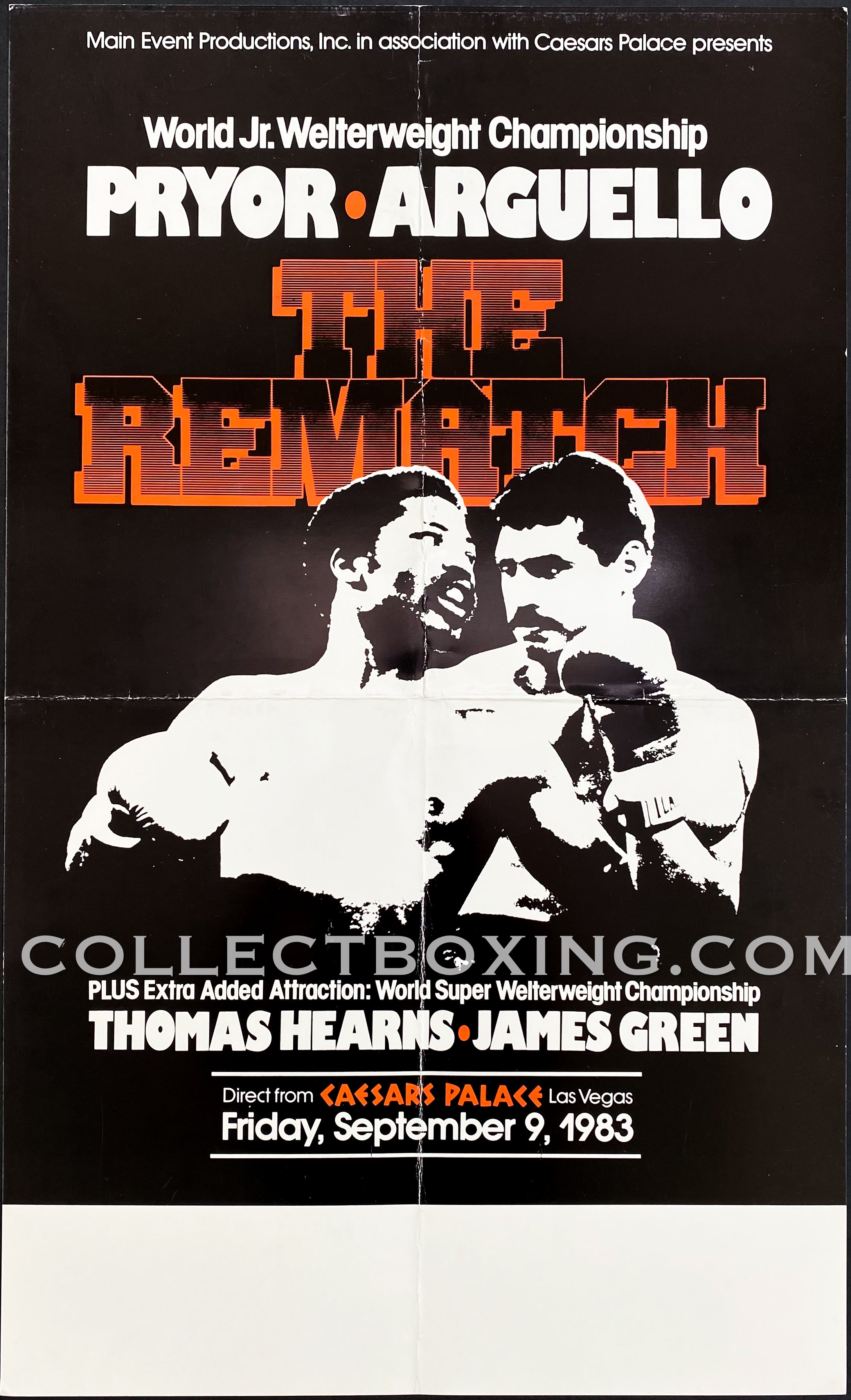This vintage promotional poster, featuring a black background with white and orange text, advertises the World Junior Welterweight Championship rematch between Pryor and Arguello on September 9th, 1983, at Caesars Palace, Las Vegas. The headline "The Rematch" is prominently displayed in large orange block letters above a high-contrast black-and-white photo of the two boxers facing each other with gloves on. Below the image, an additional attraction is noted: the World Super Welterweight Championship featuring Thomas Hearns and James Green. The poster, which shows creases indicating it has been folded, also includes the website collectboxing.com, presumably for ticket purchases or more information. The main event is presented by Main Event Productions, Inc. in association with Caesars Palace.